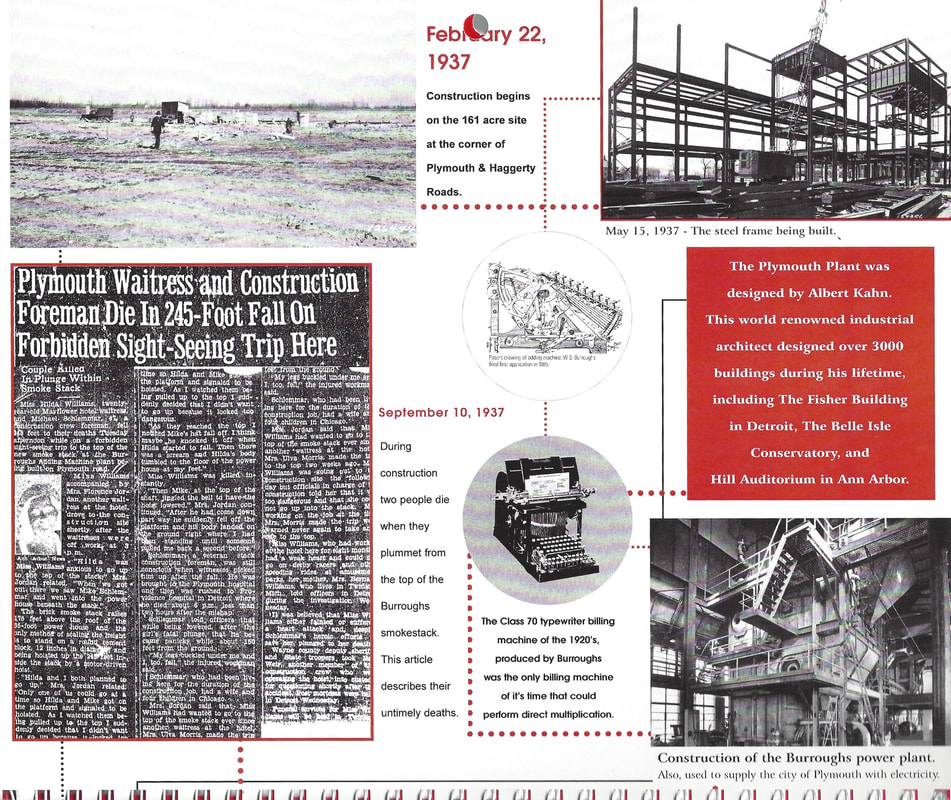This black and white print publication, accented with red spot color and in landscape orientation, appears to be an infographic or museum display detailing the construction history of the Burroughs Power Plant in Plymouth, Michigan. Central to the infographic is a depiction of the plant’s timeline, beginning with the text "February 22, 1937," marking the start of construction on the 161-acre site at the corner of Plymouth and Hagerty Roads. Adjacent to this text, on the left, is a photograph of a barren field with construction debris, while to the right, another photograph dated "May 15, 1937," shows the steel frame being erected.

Prominently featured is the name of Albert Kahn, a world-renowned industrial architect credited with designing the plant. Kahn, who designed over 3,000 buildings including the Fisher Building in Detroit, the Belle Isle Conservatory, and Hill Auditorium in Ann Arbor, is highlighted in a red text box with white text.

Further details include a notable diagram of the Class 70 typewriter billing machine from the 1920s, lauded for its ability to perform direct multiplication. This diagram is centrally located with accompanying explanatory text.

A tragic event during the construction is also memorialized. A newspaper scan in the bottom left corner, headlined “Plymouth Waitress and Construction Foreman Die in 245-Foot Fall on Forbidden Sightseeing Trip Here,” recounts the deadly incident on September 10, 1937, when two individuals fell from the smokestack, their deaths starkly noted in the display.

Complementing these textual and graphic elements is a photograph in the lower right captioned “construction of the Burroughs Power Plant,” depicting the interior stages of the build with visible metal supports and scaffolding. The overall style of the infographic blends photographic illustration and representationalism to convey a comprehensive historical narrative.